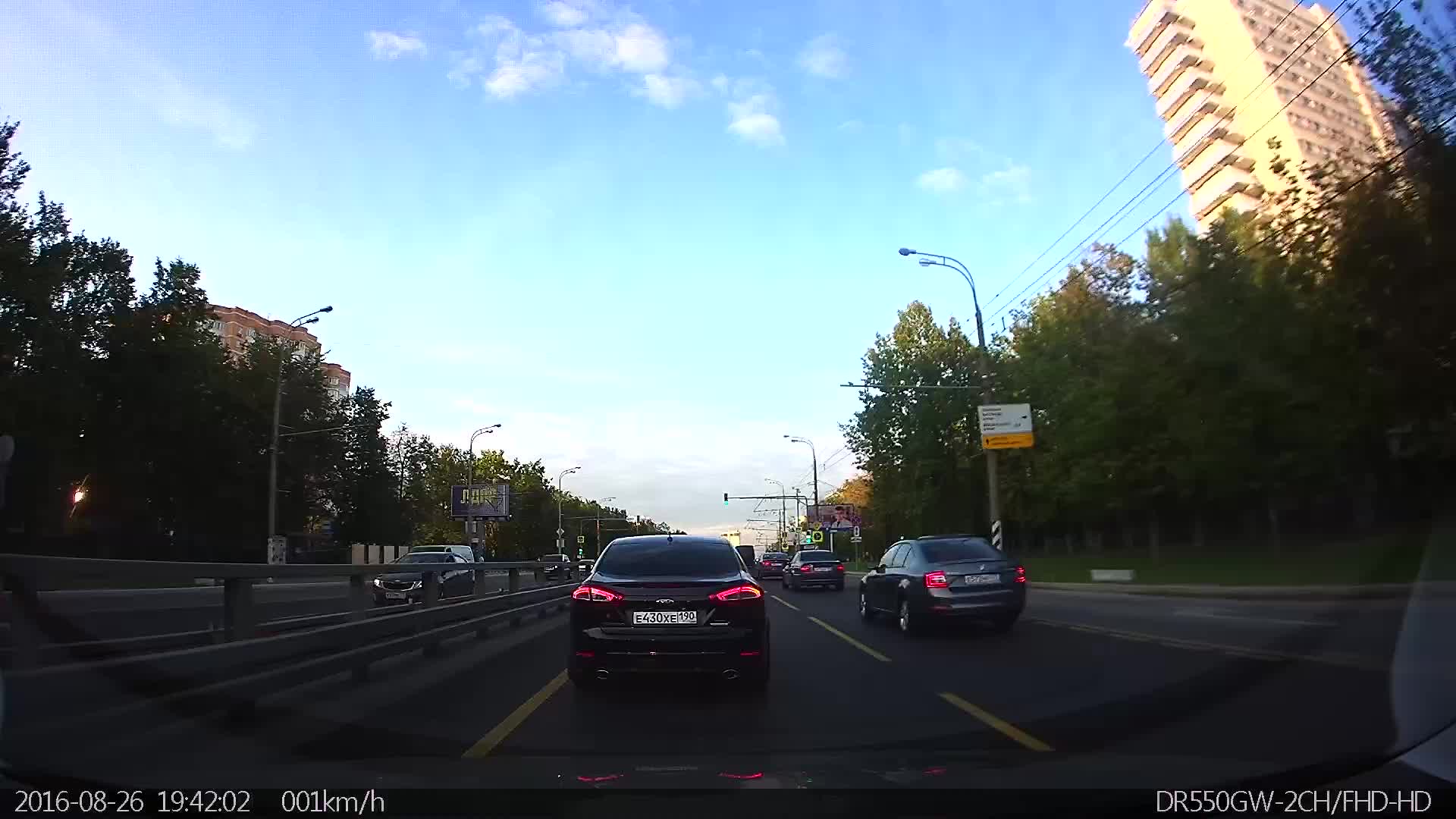This image is a still photograph, likely captured by either a dash cam or a camera held by a person inside a vehicle, looking through the front windshield. The timestamp on the bottom of the image indicates it was taken on August 26th, 2016, at 19:42:02, and the car is trailing at a leisurely speed of 001 kilometers per hour, hinting at slowing or stopping traffic. The model noted in the image, DR550GW-2CH / FHD-HD, suggests a specific dash cam model.

The scene captures a large, wide road with a barrier dividing traffic moving in opposite directions. The vehicle is in the left lane of a two-lane road direction. Various cars ahead and in the adjacent lane have their brake lights illuminated, indicating deceleration or a halt. The road features yellow markings, characteristic of its dark grey-blackish gravel.

On both sides of the road, tall trees are visible, framing the street. Beyond these trees, high-rise apartment buildings rise, especially prominent on the right side. On the left side, another building can be faintly seen peeking above the tree line. The sky is a vibrant blue with a scattering of white clouds, suggesting a bright sunny day, although the surrounding area below remains relatively dim in comparison. The diminishing light levels further indicate either dusk or early morning. Additionally, visible street signs and license plates imply the setting is outside the United States, featuring characters that are not in English.